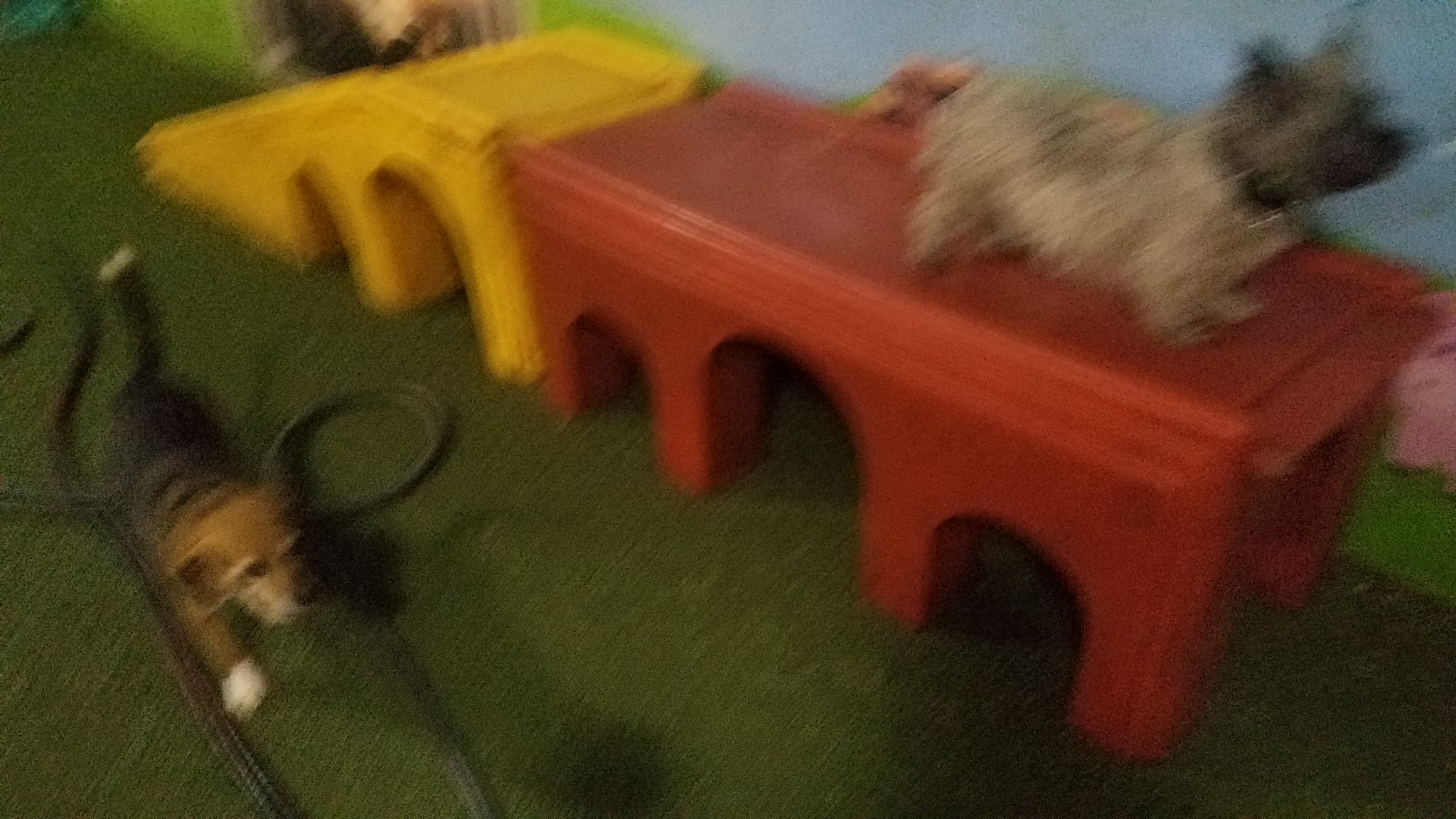In this slightly lower resolution and somewhat blurry, grainy image, there are two small dogs positioned on different parts of the frame. The dog on the left has white paws, light brown fur around its face, black fur covering its back, and a tail tipped with white. The dog on the top right sports a darker gray, shaggy head and a light gray body. This second dog is standing on colorful daycare play furniture, which features arches, bridges, and a yellow slide. Meanwhile, the dog on the left navigates around some hoses. The setting boasts a dark green carpet and a possibly painted wall in the background, indicative of an indoor daycare environment for pets.